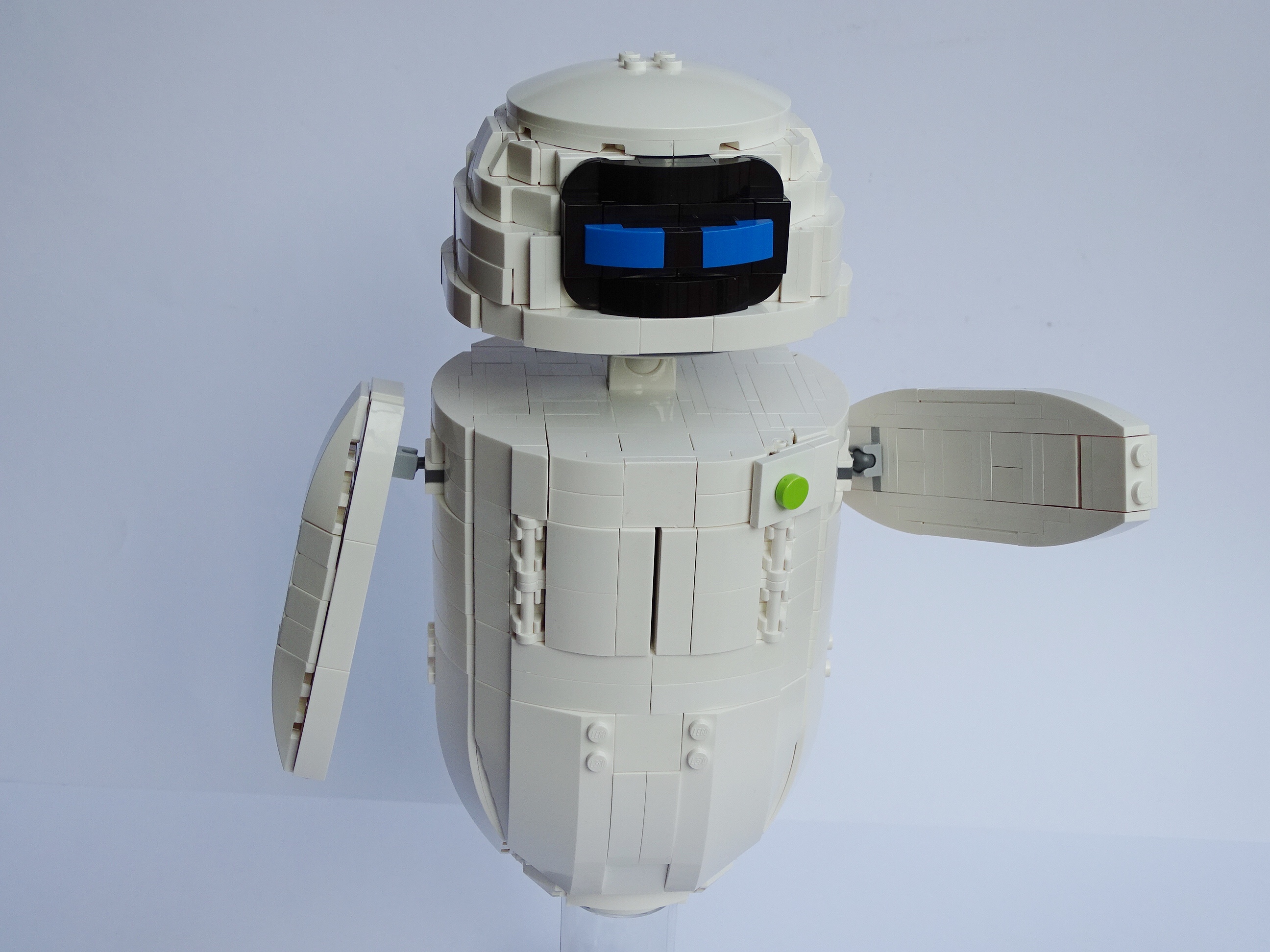The image depicts a small, intricately designed Lego robot. Constructed primarily out of white Lego pieces, the robot features two blue Lego pieces forming an LED-like screen for its eyes, and a black piece beneath it, giving the impression of a facial screen display. The robot has two maneuverable arms, each capable of 360-degree rotation, with the left arm stretched outward and the right one pointing diagonally downward. A notable detail includes a Lego part with a green button. Although the robot lacks legs, it has a rounded base, reminiscent of R2D2 from "Star Wars." The robot is set against a light gray background and is positioned centrally, suggesting it was placed on a table by its creator for display purposes. The image includes various colors such as lime green, white, black, blue, and light blue, contributing to the detailed and playful aesthetic of this Lego creation.